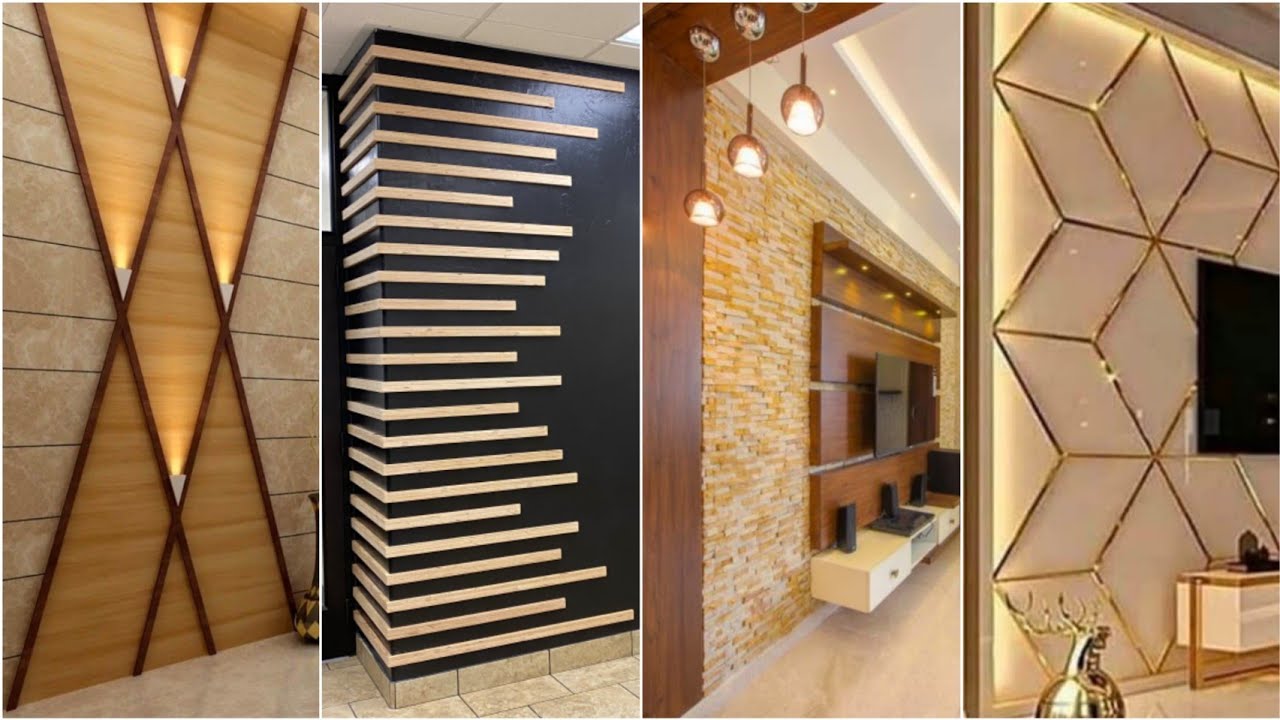This image depicts a stylish collage of four vertical photographs showcasing different wall treatments within a luxurious and high-tech home. The far-left panel features a wall adorned with horizontally sliced stone slabs intersected by two striking vertical gold X patterns, accompanied by conical white light sconces that illuminate the wood-paneled interior. Moving to the second panel, we see a black rectangular pillar corner embellished with horizontal wooden strips of varying lengths, creating a dynamic visual contrast against the dark background. The third panel reveals a living room wall with a pale gold and cream brick facade wrapping around an entertainment center. This setup includes recessed ceiling lights, hanging pendant lights, and a large dark-stained wood panel that houses a mounted large-screen TV, accompanied by a high-tech stereo system on a white marble floor with gray accents. The final panel behind another TV set showcases an intricate geometric design of large, connected diamond shapes forming a hexagonal snowflake pattern, constructed with brass or gold-colored metal rods, adding a delicate touch of elegance to the modern decor.